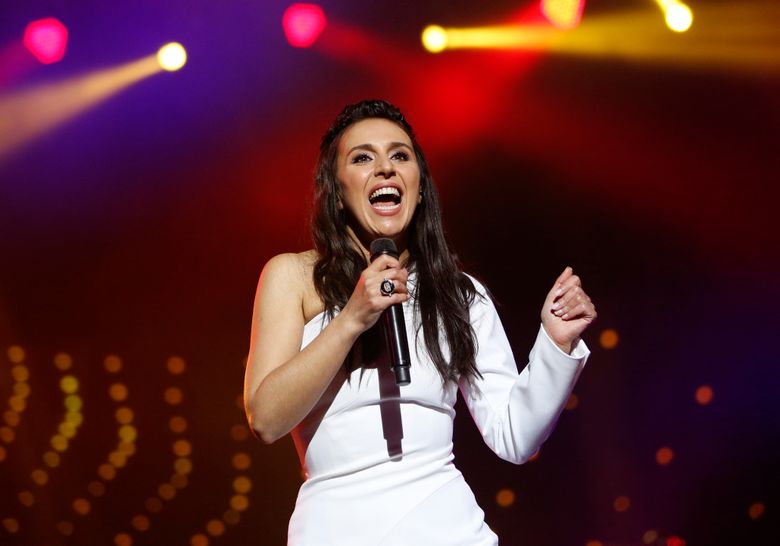Against a dramatic backdrop of blurred red, pink, and yellow lights creating a vibrant yet dark ambiance, a close-up photograph captures a white woman in her 30s, possibly a singer, mid-performance on stage. The background is a mix of dark hues and bright spotlights from the ceiling, with numerous small dots of pink and yellow lights contributing to the dynamic atmosphere. The performer, with long brown hair framing her face and covering her chest, is clad in a striking white dress that features a unique design: one shoulder is covered with a sleeve extending to her hand, while the other shoulder is bare. Her makeup is meticulously done, highlighting her beautiful eye makeup, black mascara, and light lipstick. With an expressive open mouth revealing straight white teeth, she appears to be passionately singing or talking loudly. She holds a black microphone adorned with a black ring on her right hand, facing the camera. This image captures the intensity and emotion of her live performance.